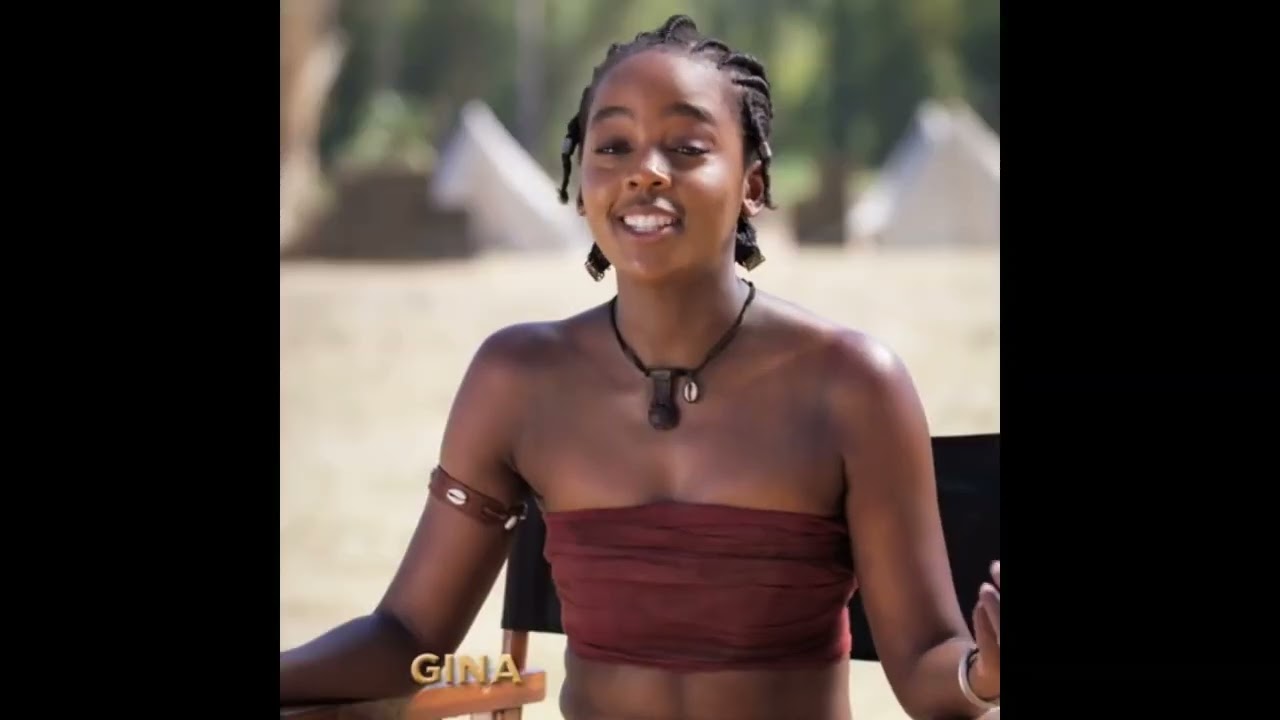The image features a young, pretty black woman named Gina, as indicated by the yellow text in the bottom left corner. She is sitting in a director's chair with wooden arms and a black back, smiling radiantly with her eyebrows raised and eyes lit up, suggesting she may be singing or expressing joy. Gina is dressed in a reddish maroon tube top and accessorized with a leather band and a watch on her arm, along with a distinctive necklace that seems to have an African or puka shell design. Her hair is styled in short cornrows pulled back. The background is blurred, showing what appear to be white tents and brown objects, adding an ambiguous yet intriguing atmosphere to the scene, possibly indicating she is on the set of a movie, television show, or reality show like Survivor. The photo itself is presented in a landscape orientation with thick black borders on either side, giving it a square-like appearance.